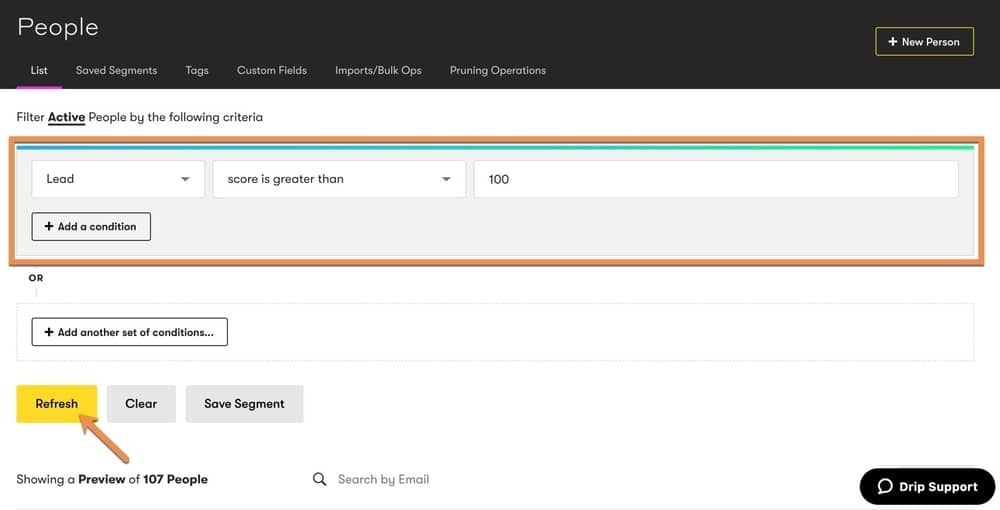This image showcases a webpage interface with a clear organizational structure. At the top, a black bar spans the width of the screen. On the left side of this bar, there's the text "People," and on the right side, there is a square icon featuring a plus sign and a person. 

Below this bar are several tabs arranged horizontally, labeled from left to right as: Lists, Saved Segments, Tags, Custom Fields, Import/Bulk Ops, and Pruning Operations. Beneath these tabs, there is a section titled "Filter active people by the following criteria."

This section contains a brown-bordered area divided into three segments. The first segment on the left specifies "Lead score is greater than," followed by the numeric value "100." Below this criterion, there's a button labeled "+ Add a condition."

Further down, the word "or" is displayed, providing an option to specify alternative criteria. Below this word, there's another button reading "+ Add another set of conditions."

At the bottom of the brown-bordered section, three buttons are aligned horizontally from left to right: Refresh, Clear, and Save Segment.